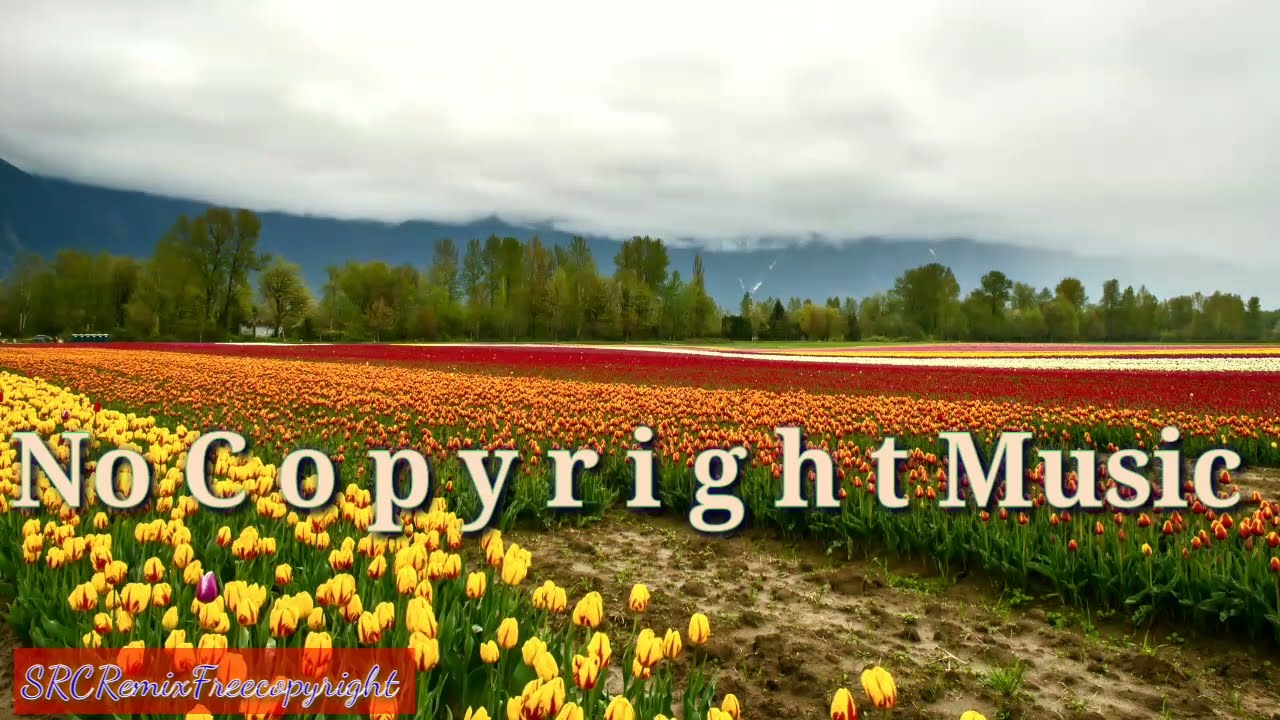The image captures a vivid, expansive field of meticulously planted flowers, arranged in rows of different colors which span across the majority of the scene. Dominating the foreground, there is a prevalent mix of bright yellow flowers, succeeded by bands of orange and red flowers, creating a striking gradient effect. On the lower left corner, a transparent red box boldly displays the text "S.R.C. Remix Free Copyright" in legible cursive blue. The flowers stretch far into the distance, with an interruption of a small, empty dirt section on the lower right. As the eye moves towards the horizon, a line of lush, green trees demarcates the boundary of the flower field, standing beneath a sky heavily blanketed with white clouds, allowing mere glimpses of blue. The entire scene seems slightly enhanced, giving it an almost surreal vibrancy.